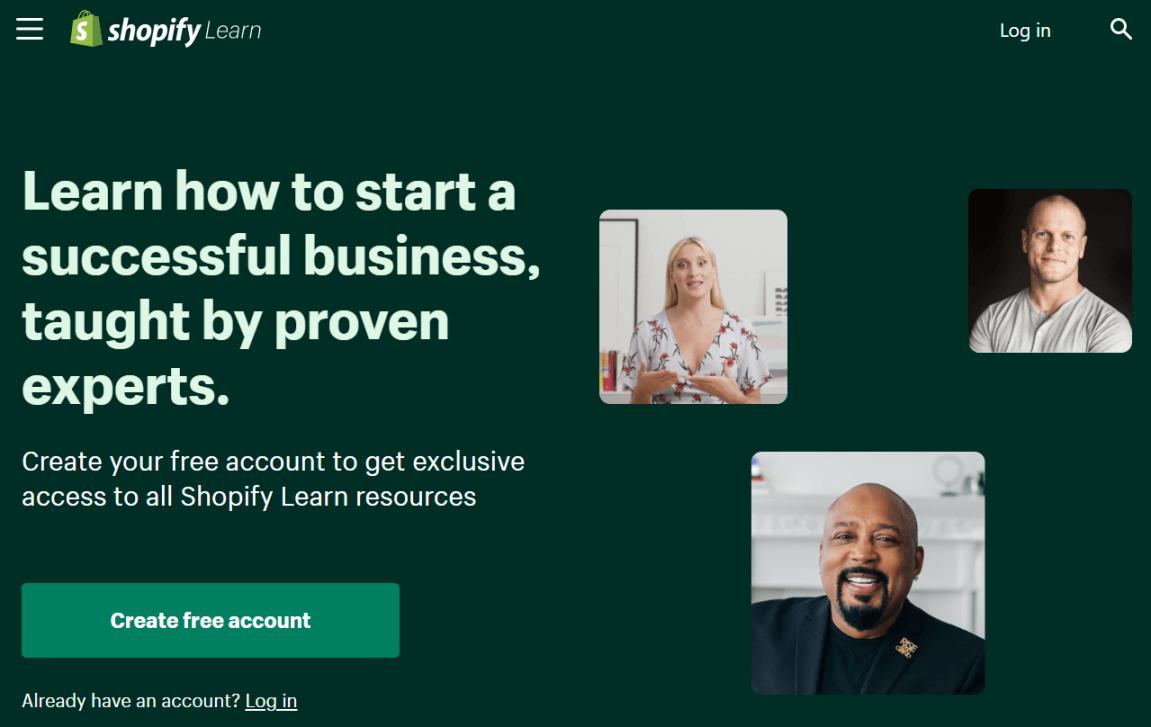The image features a vibrant green background that highlights three distinct portraits of individuals. On the left, there is a white female with blonde hair, wearing a white dress adorned with floral patterns. Her background is predominantly white, creating a soft contrast with her attire. 

In the center, there is a white male with a primarily black background. He is bald, with a muscular build and a well-defined jawline, complementing his happy and friendly smile.

On the right, there is a black male, identifiable as Damon John from "Shark Tank." He sports a neatly groomed beard and is bald, dressed in a sharp black suit accessorized with a pendant. He also exudes a warm smile.

To the left of these portraits, there's a text overlay inviting viewers to "Learn how to start a successful business taught by proven experts." It prompts users to "Create your free account to get exclusive access to all Shopify Learn resources," with options to create a free account or to log in if they already have one.

At the top of the image, a banner reads "Shopify Learn," accompanied by a login button and a magnifying glass icon for search functionality. To the left of the Shopify Learn logo, a familiar three-line menu icon is visible, indicating additional navigation options.